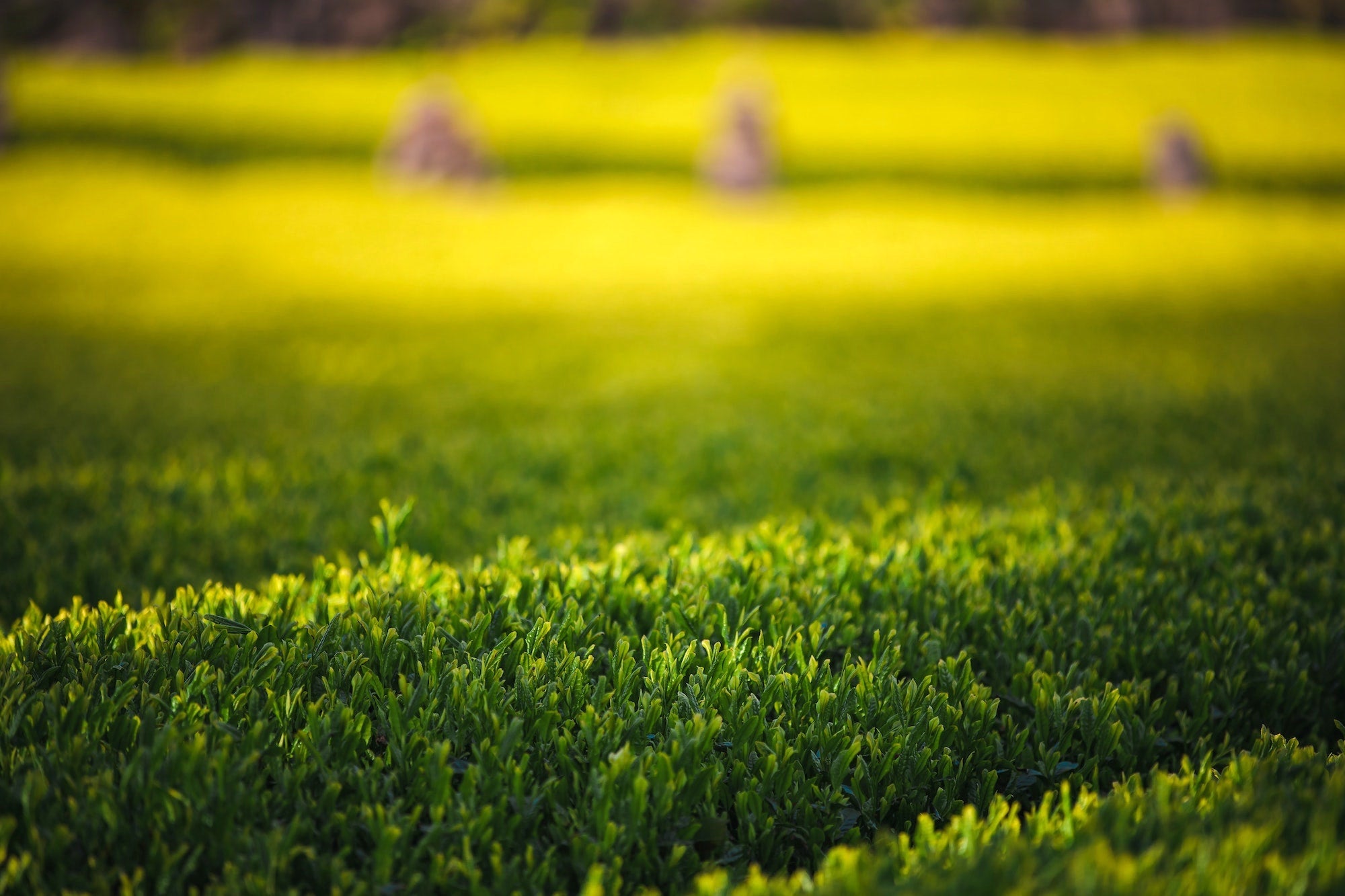The photograph is a horizontal, professional-grade image showcasing a vibrant outdoor scene. In the foreground, a meticulously captured row of green hedges, varying slightly in height and maintaining a somewhat untrimmed appearance, commands attention. The viewer's perspective is from the top of these hedges, highlighting their lush texture and deep green coloration. As the eye moves towards the background, the image becomes progressively blurrier, transitioning into a softer landscape filled with vivid colors.

In the mid-ground, the hues shift from the rich green of the hedge to lighter green tones, indicative of either a different type of vegetation or a field. This area features three distinct groups of purple flowers, positioned strategically to the left, center, and right, adding splashes of contrasting color. Beyond this, the scene transforms into a field dominated by golden-yellow flowers, suggesting an expanse of crops or wildflowers.

Further back, three brown, cone-like structures punctuate the yellow field, possibly resembling haystacks or other agricultural elements. The image finishes with a very blurred background, hinting at the edge of a wooded area or another indistinct natural boundary. This masterfully blurred effect enhances the overall depth and focus of the photograph, making the detailed foreground stand out more prominently against the softer, colorful backdrop.